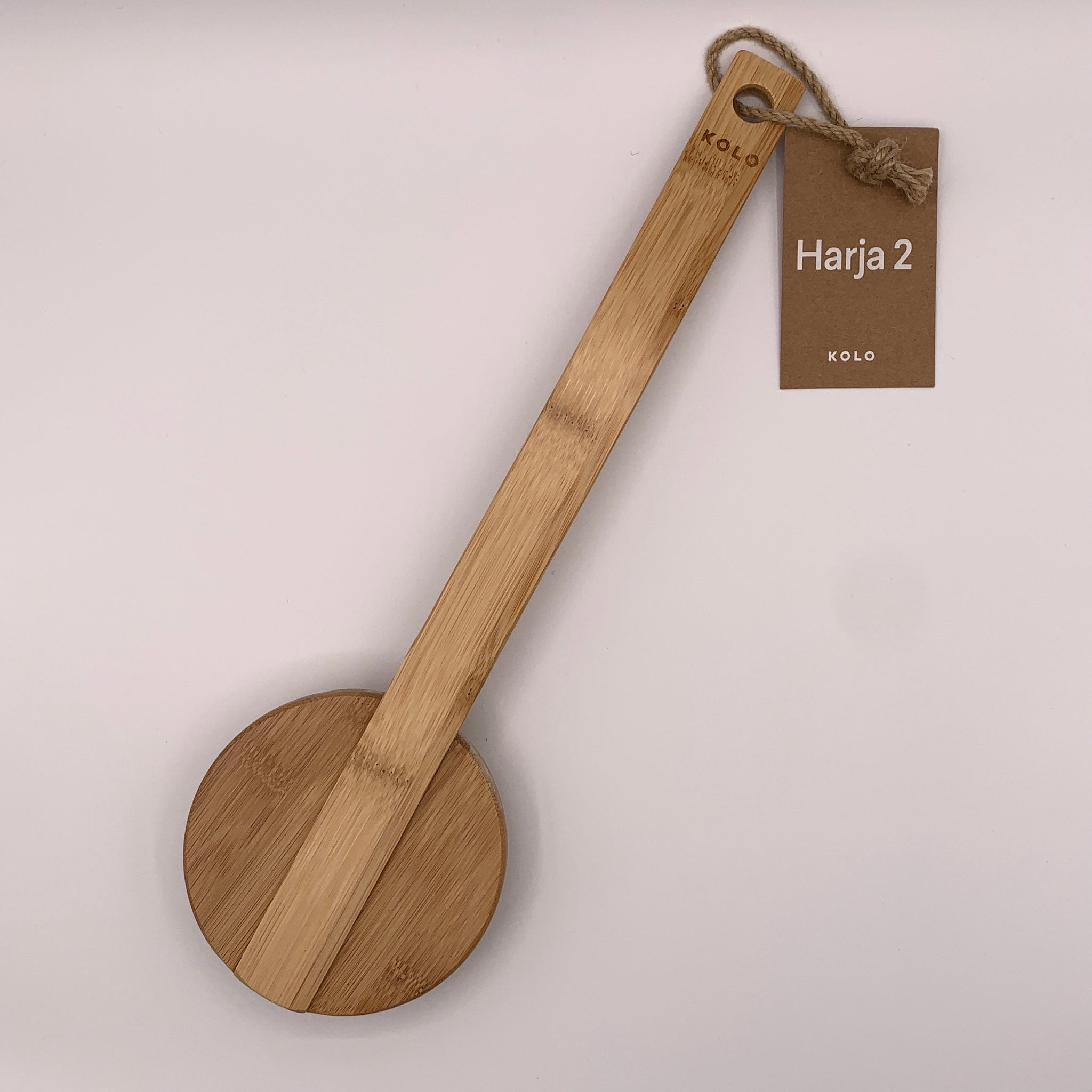This image showcases a wooden tool, possibly a back scrubber or another bath accessory, set against a light gray background. The tool's design features a long, vertically-aligned rectangular handle made of a light to medium brown wood, which could be bamboo, displaying a distinctive grain pattern. The handle is angled slightly, with the top leaning right and the bottom left. 

At the bottom of the handle, there is a deeper brown circular wooden element, which may serve as a part of its functional design. The handle extends upward and culminates in a circular cutout at the top. Through this cutout, a dark brown rope is threaded, suspending a dark brown rectangular paper tag. The tag bears the inscription "HARJA2 K-O-L-O" in white text, which is also engraved just below the circular cutout on the handle. 

The overall appearance suggests it could be a premium bath accessory, perhaps found in specialty stores such as Bath & Body Works.